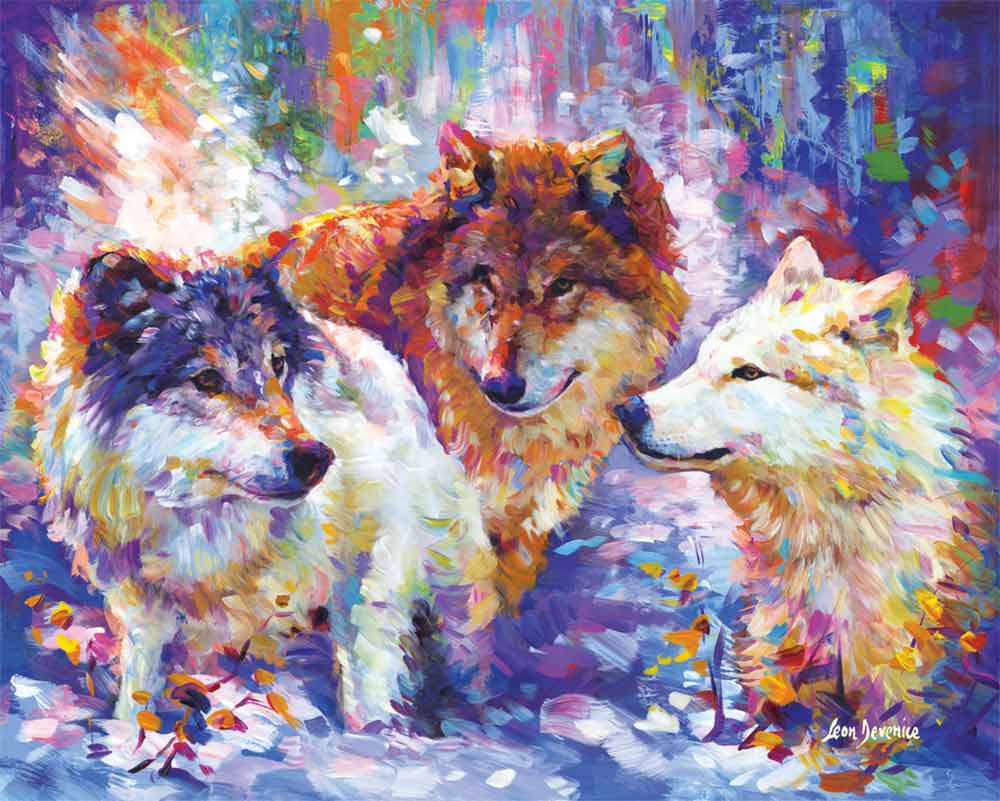This highly stylized Impressionist painting by Leon Javinis features three wolves set against a vibrant, multicolored background. The backdrop bursts with various hues including purples, blues, greens, oranges, whites, reds, pinks, and burnt orange. The painting's lower section is dominated by shades of white, gray, blue, and light purple, suggesting a winter landscape with snow. 

In the center foreground, three distinct wolves draw the viewer's attention. The leftmost wolf has a white body with a gray head and purple-tinted fur on its ears. The central wolf stands proud with a dense brown fur coat and pointed ears, slightly tilting its head to the left. The rightmost wolf, predominantly white with pointed ears and a black nose, features a colorful mix of pinks, purples, blues, greens, and yellows running through its fur. The wolves appear to be engaging with each other, their poses creating a sense of interaction amidst the explosion of colors that fills the painting.